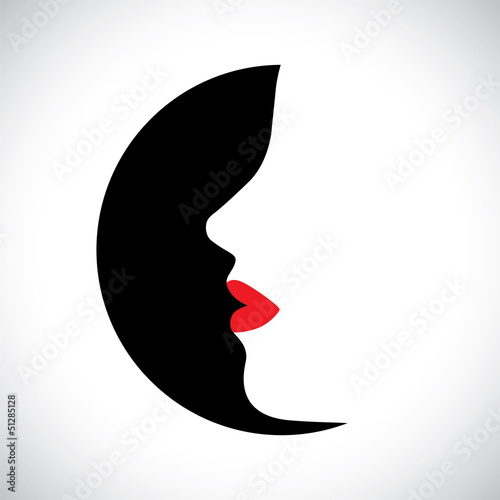The image features an abstract depiction that blends multiple visual interpretations. Set against a light gray or white background, the central focus is on a black semicircle resembling a crescent moon or a circular disc. Intriguingly, the silhouette of what appears to be a woman's face is seamlessly integrated into this black shape, showing her chin, nose, and forehead as if cutting into the moon-like crescent. The red lips, which could also be perceived as a heart turned sideways, add a striking contrast to the image. This duality creates an optical illusion where the viewer might see either a black crescent moon encroaching on a female profile or a simple face with vividly red lips against the black crescent. Overlaid faintly across the entire image are diagonal watermarks saying "Adobe Stock," with a clearer "Adobe Stock" and a number, 51285128, located at the bottom left corner, indicating copyright.